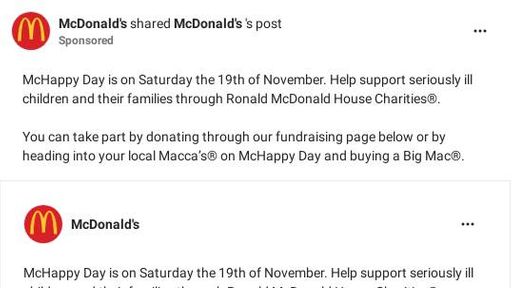Sponsored Post: McDonald’s Invites Support for McHappy Day

In this sponsored post shared on Twitter, McDonald’s is promoting McHappy Day, set for Saturday, November 19th. The post features the iconic McDonald's logo on the left, with the familiar golden arches on a red background. McHappy Day is an initiative aimed at supporting seriously ill children and their families through the Ronald McDonald House Charities. 

To participate, individuals can donate via the provided fundraising page or by visiting their local McDonald's, commonly referred to as "Maccas." Purchasing a Big Mac on this day will also contribute to the cause. 

This post includes a mix of sponsored content, characterized by a white background and black text, and subsequent reposts to further spread the message. Join the effort to support families in need by contributing to McHappy Day on November 19th.

[Note: The repost mentioned it discussing the effectiveness of the charity.]